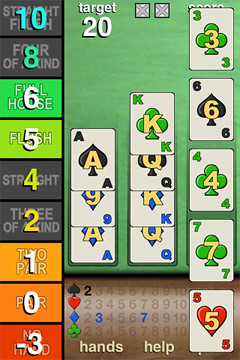This image depicts a detailed scene of a card game being played on a smartphone, displayed in landscape mode. On the left side of the screen, a vertical column features a series of colored squares with numbers and associated poker hand descriptions: a gray square marked '10' labeled 'Straight flush,' another gray square marked '8' labeled 'Four of a kind,' a lime green square marked '6' labeled 'Full house,' a different green square marked '5' labeled 'Flush,' a gray square marked '4' labeled 'Straight,' another gray square labeled '3 of a kind,' a light orange square marked '1' labeled 'Two pair,' a dark orange square marked '0' labeled 'Par,' and a red square marked '-3' labeled 'No hand.'

Dominating the right side of the image, the words "Target 20" are displayed in white over a green background, which serves as the playing field. Various cards are laid out on this field, including the 3 of Clubs, 6 of Spades, 4 of Clubs, 7 of Clubs, and 5 of Hearts, which sits upon a brown overlay with illuminated numbers and symbols. Additional rows feature cards such as the King of Clubs, Queen of Spades, King of Diamonds, Queen of Diamonds, Ace of Spades, 9 of Diamonds, and Ace of Diamonds. The layout suggests a solitaire or unique version of poker, with a mix of card ranks and suits displayed on the screen.